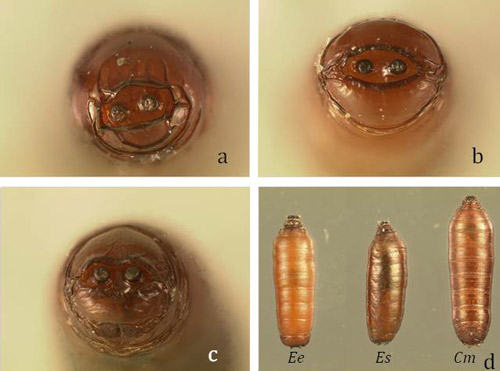The photograph consists of four close-up images labeled A, B, C, and D, depicting the developmental stages of an insect, possibly a weevil. Images A, B, and C focus on the insect's face at different stages of emergence from its shell or cocoon. The insect's face is brownish-red with visible black eyes, giving it an unsettling appearance resembling a blister on human skin. Its body transitions to a goldish-red color as it emerges. Image D, in the bottom right, shows three specimens at various life stages labeled E (bronze-colored), ES (darker brown), and CM (a mix). The images provide a disturbingly detailed view of the insect's morphology through its lifecycle. Different colors and labels indicate distinct growth phases, offering a detailed scientific study of the insect's development.